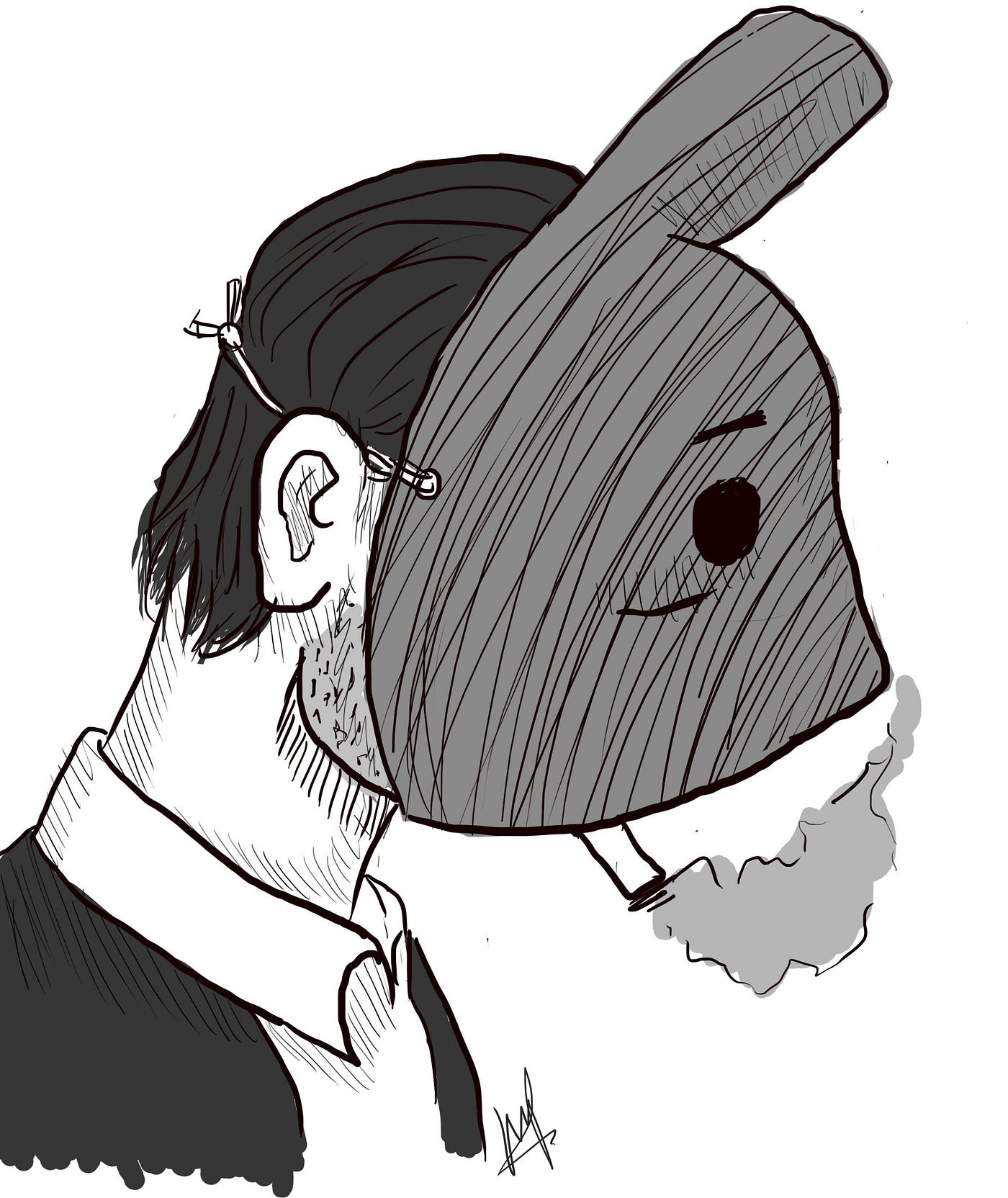The image is a black-and-white pencil sketch of a man wearing a half-mask resembling a bunny rabbit, complete with tall ears and sad eyes. The mask is tied behind his head with a visible string. The man has short, dark hair stopping just below his ears, and a noticeable five o'clock shadow. He is dressed in a white collared shirt under a dark sweater or jacket. A cigarette protrudes from his mouth beneath the mask, with grey smoke drifting upward. The sketch features intricate line work and shading, with the artist's signature at the bottom, though it is unclear.